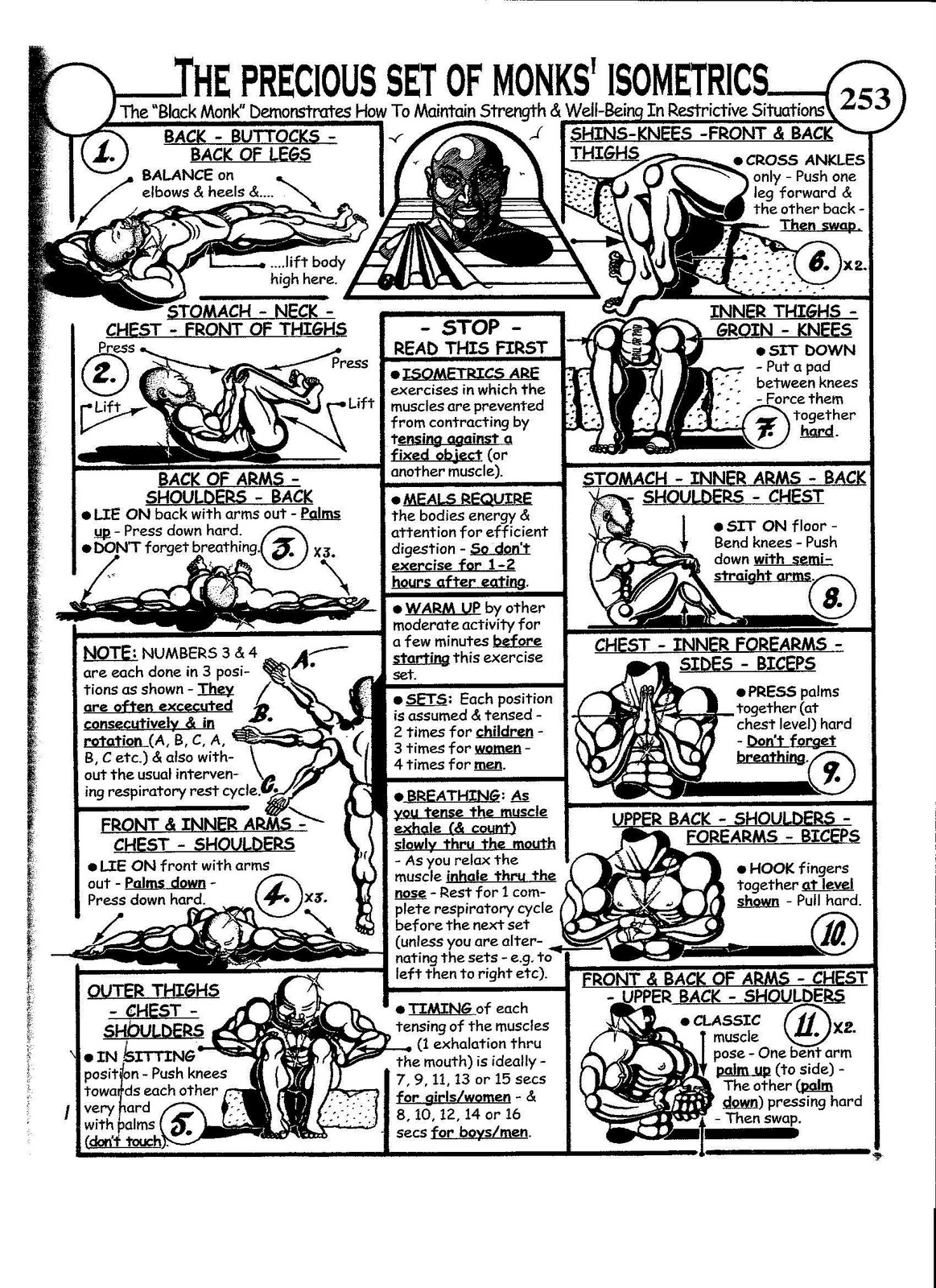This detailed black-and-white infographic serves as a compact and dense guide titled "The Precious Set of Monks Isometrics," identified by the circle number 253 on the top right corner. It is designed to help maintain strength and well-being in restrictive situations, as demonstrated by "The Black Monk." 

The infographic is divided into 11 numbered boxes, each showcasing a different isometric exercise along with detailed instructions. The first exercise features a male figure clad in shorts, lying on his back with his hands behind his head. The caption reads: "Back, Buttocks, Back of Legs - Balance on Elbows and Heels, and Lift Body High Here."

At the very top center of the infographic, an illustration of a smiling monk invites viewers to "Stop, Read This First." This section provides essential information on understanding isometrics, including guidance on necessary meals, warm-ups, sets, breathing techniques, and timing.

The detailed visual and textual content aims to systematically guide the viewer through a series of exercises, each meticulously explained and illustrated, to enhance physical fitness even in limited environments.